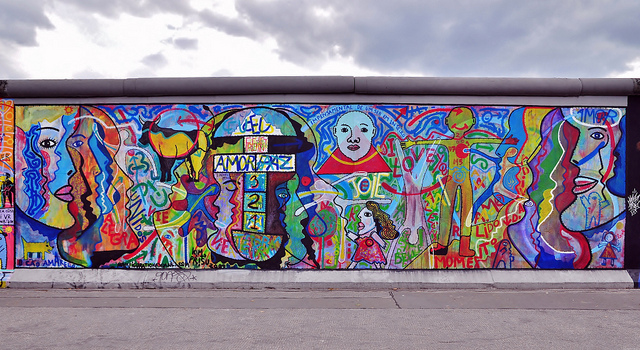The photograph captures a vibrant mural painted on a long flat wall, set against a cloudy gray-blue sky. The mural, adorned with an array of bright, neon-like colors including blues, reds, greens, and yellows, features various abstract and caricatured human faces. The left side is populated with multi-colored faces, and other prominent illustrations include a bald figure with a red collar, a female figure in a red dress with dark curly hair, and a stick figure in yellow. A distinctive hopscotch design, centrally located, bears the words "Amor Paz" and the numbers "3 2 1". Additional phrases such as "I love you" and "JOIE" are inscribed throughout the mural, along with numerous other letters that do not form coherent words. The mural's chaotic lines and myriad of colors create a captivating and eclectic visual experience that stands out amid the otherwise muted surroundings.